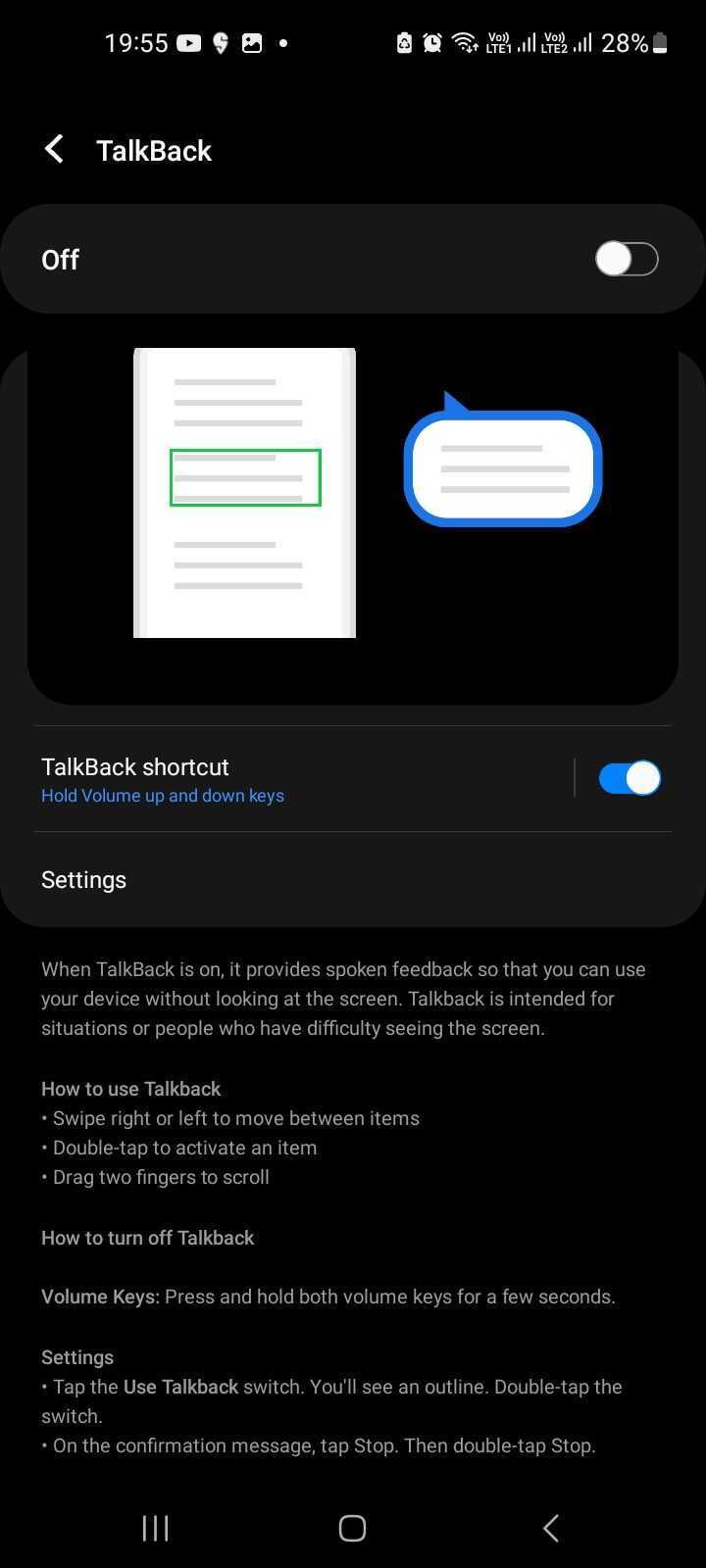This image showcases a smartphone screen displaying the accessibility settings for the "TalkBack" feature. The background of the device is black, with various icons situated at the top. On the top left, the current time is shown as 9:55, followed by the YouTube and Gallery icons. On the top right, the icons for battery saver, alarm, WiFi, dual SIM status, and battery life at 28% are displayed, all in white.

The main focus of the screen is the TalkBack settings. "TalkBack" is written prominently in white, with a toggle switch to its right, which is currently off (white). Below this, there is a rectangular overlay resembling a piece of paper with grey lines and a green border. A blue speech bubble with a white interior and grey text explains the functionality of TalkBack.

Further down, there is a section called "TalkBack shortcuts." The corresponding toggle is blue, indicating it is on. This section describes that holding the volume up and down keys will activate these shortcuts. The instructions are detailed in blue text, whereas the surrounding text remains white.

The screen continues with a comprehensive explanation of TalkBack, intended for users who have difficulty seeing the screen. It highlights how to navigate the device using TalkBack, including swiping right or left to move between items, double-tapping to select an item, and dragging two fingers to scroll. Additionally, it provides guidance on how to turn off TalkBack using volume keys or the settings menu, describing each step with clarity.